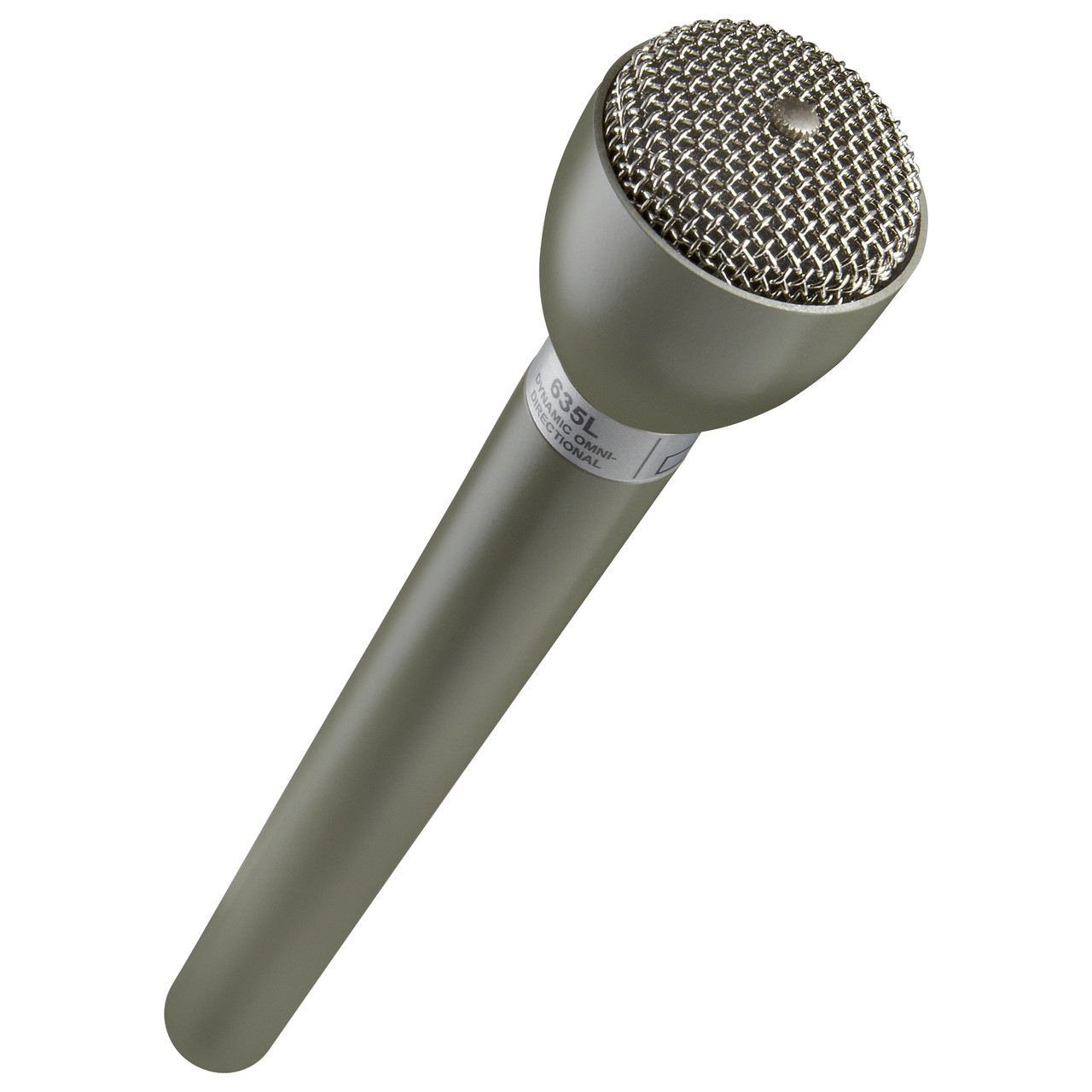This image features a single gray steel microphone with a matte finish, depicted against a plain white background. The microphone is positioned diagonally, with the handle starting at the lower left and extending upward to the top part in the upper right. Measuring approximately six inches in length, the handle is about half an inch wide at the bottom and gradually widens, reaching about an inch and a half at its widest point.

Around the top of the handle, just below the head of the microphone, there is a light gray label encircling it, displaying the text "635L Dynamic Omni Directional." The head of the microphone features a vented pattern resembling tiny diamonds or a grid, with a distinguishable round screw-like piece with grooves at the very center.

Overall, the microphone is characterized by its sleek, platinum-gray appearance, emphasized by the contrast of the lighter gray label around its handle, making it a striking and detailed portrayal of a classic audio device.